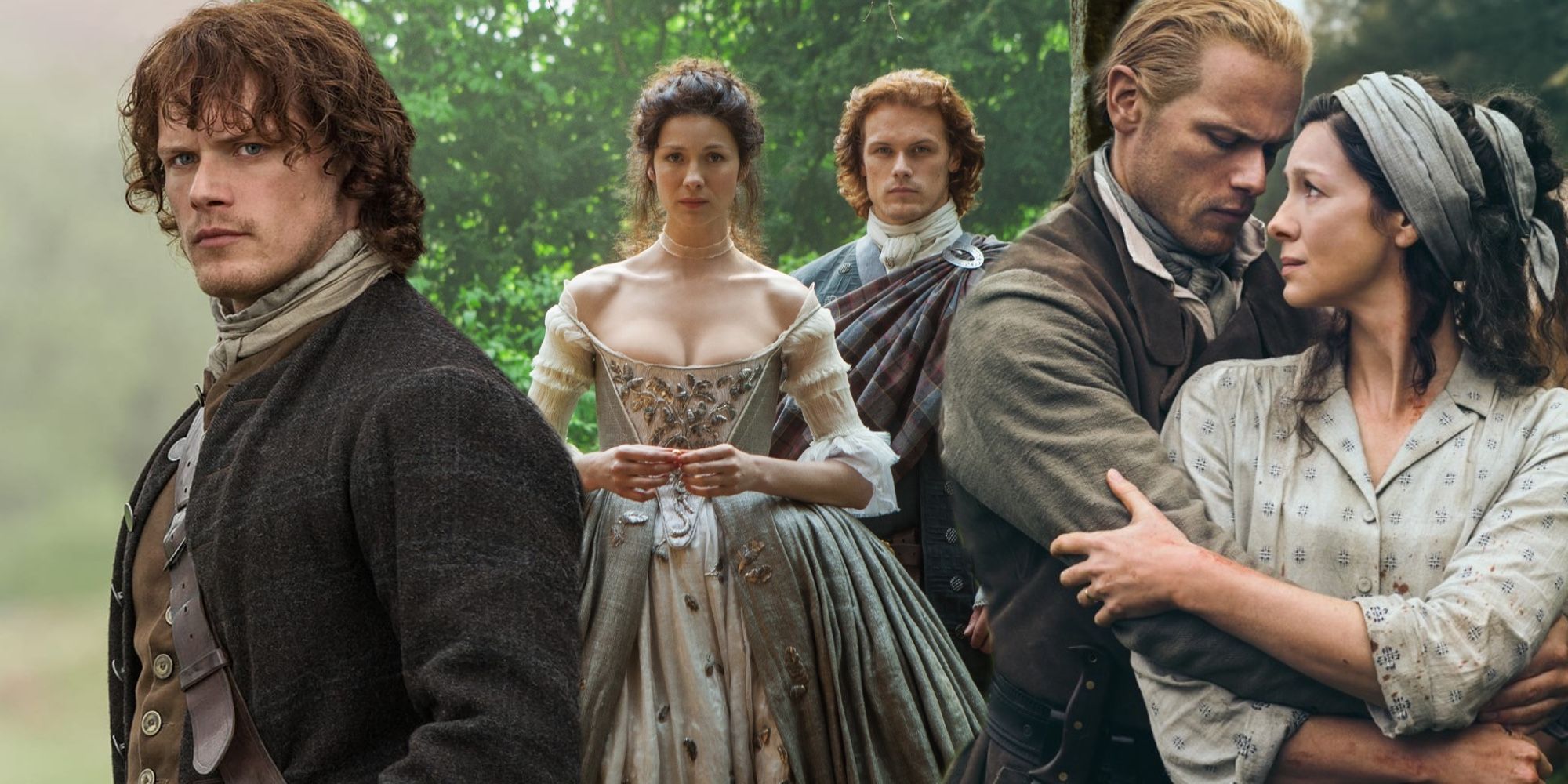The image is a meticulously composed photograph, likely photoshopped, featuring five people in early 20th-century attire, potentially from the 1910s to 1920s. The scene evokes the look of a period movie or a historical reenactment. In the center, a woman with dark, styled hair stands prominently, wearing an elaborate peasant gown with intricate embellishments, suggesting some degree of wealth. She stares directly at the camera, her lace necklace adding to her refined appearance. Beside her is a man with long reddish hair, draped in what appears to be a Scottish cape; he too gazes intently at the camera. Behind them, the backdrop shifts to soft-focus foliage and large green trees, contributing to the vintage ambience.

To the left, a man in a dark gray suit with long brown curly hair stands solemnly, a stern expression on his face. He faces to the left but seems caught in contemplation. He wears a wool jacket and has a bag slung across his torso.

On the right side of the image, another couple is depicted in an emotionally charged pose. The man, with slicked-back hair, has his arms wrapped protectively around a woman. She clutches his arm and gazes distantly, her dark hair pulled up and adorned with fabric. She wears a light-colored button-up shirt with a pattern, adding depth and texture to her look.

All characters appear slightly worn and dirty, enhancing the historical authenticity of the scene. The layered clothing and emotional expressions contribute to a tableau that feels both intimate and richly detailed.